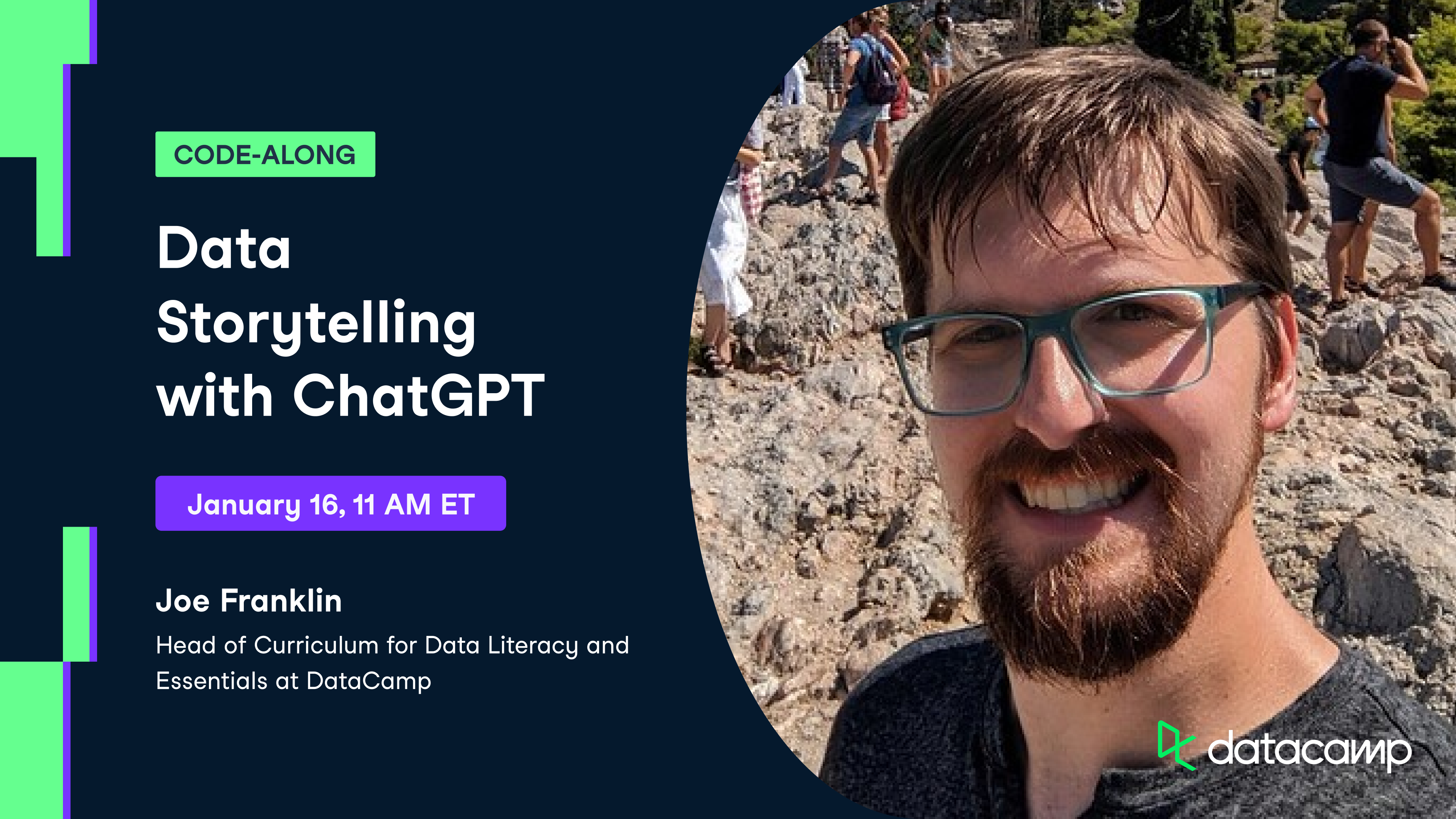**Website Event Page: Data Storytelling with Chat GPT**

The webpage features a blue background with various visual elements and text. On the right side, there is a circular image with a photo of a man in a natural outdoor setting. The man has green glasses, a beard, and a mustache, and he is smiling. Behind him, people are dressed in warm-weather attire such as shorts, t-shirts, and sandals, carrying backpacks and appearing to be on a hike. The background includes rocky terrain and trees. The photo is branded with the "Data Camp" logo in the bottom right corner.

On the left side of the page, green and purple markings add visual interest. A green box contains the text "Code Along", while a purple box below it has white letters that read "Data Storytelling with Chat GPT". The event details are noted as taking place on January 16 at 11 a.m. ET. Beneath this, additional text introduces Joe Franklin, who is the Head of Curriculum for Data Literacy and Essentials at Data Camp. 

Overall, the page effectively combines imagery and text to promote the upcoming event, making it visually appealing and informative for visitors.